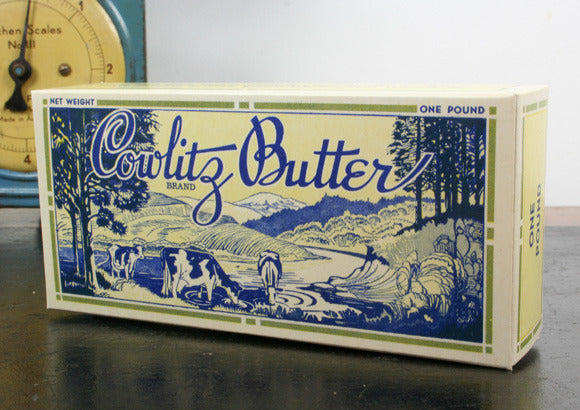The photograph captures a vintage-style box of Cowlitz Butter, prominently placed on a wooden table. The butter box features a nostalgic 1940s script font stating "Cowlitz Butter" and indicates a net weight of one pound. Dominated by blue and yellow colors, the rectangular package showcases an old-timey illustration of three cows drinking from a stream, surrounded by rolling green hills and trees, with mountains in the backdrop. The illustration is bordered by a green strip, adding a further touch of quaint charm. In the background, old-style kitchen scales enhance the vintage ambiance, while the smooth black surface and a light blue clock on a white wall provide subtle modern contrasts. The vivid, modern photograph style ensures the butter box remains the focal point of the image.